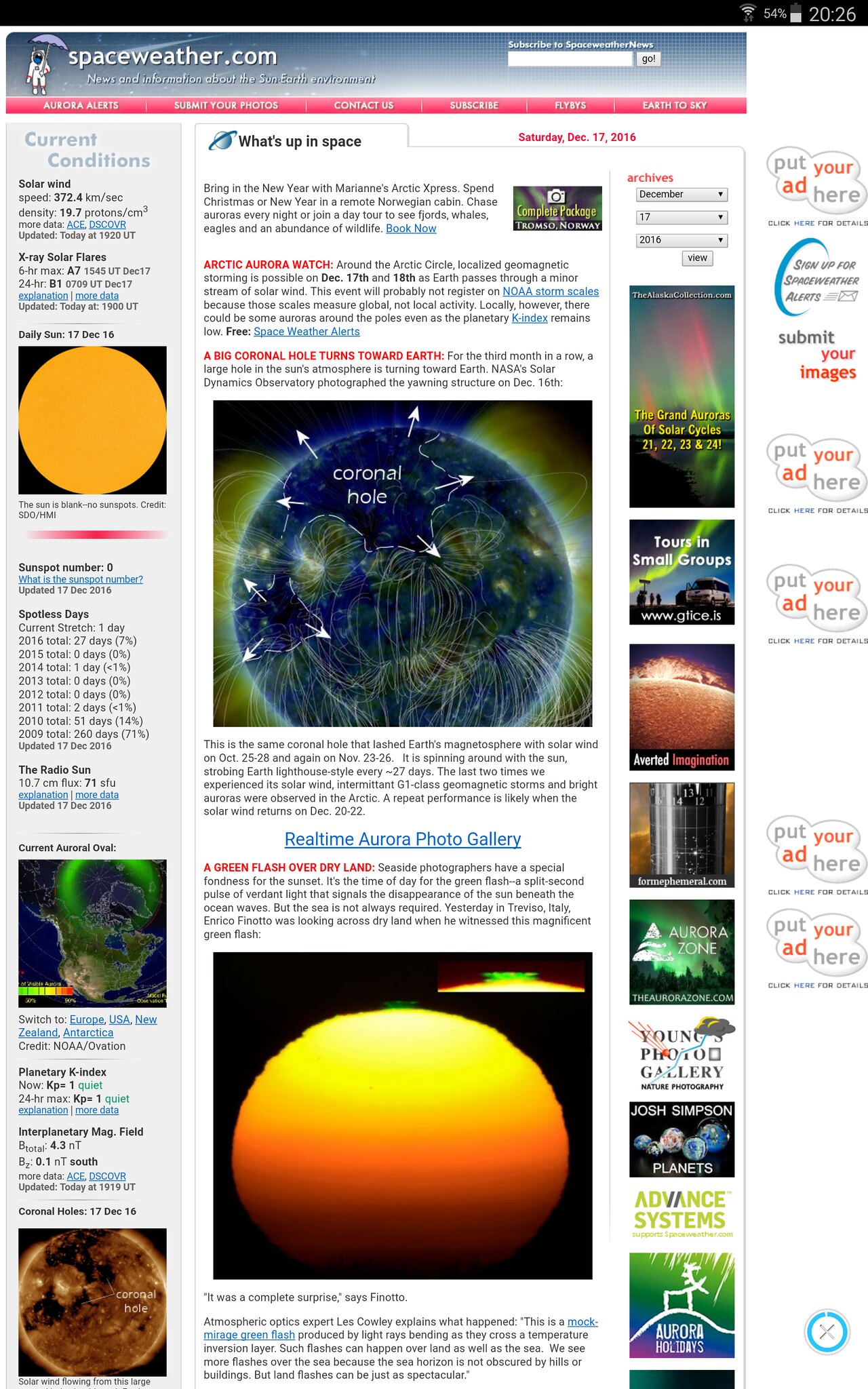The image is a detailed screenshot of the website "spaceweather.com," likely viewed on a mobile device, as suggested by the Wi-Fi signal, battery icon at 54%, and the time stamp 20:26 in the upper right corner against a black bar. Below this, the website's name "spaceweather.com" is prominently displayed in white letters on a blue to gray gradient bar. Beneath, the navigation menu includes "Aurora Alerts," "Submit Your Photos," "Contact Us," "Subscribe," "Flybys," and "Earth to Sky," marked by a thin purple line with white text.

The screenshot captures various columns of informational content. On the extreme left, a vertical column invites advertisements. The next column details current space weather conditions, featuring images of the sun and Earth, including a topographic map of the USA with a green haze and a daily update dated December 17. The central column highlights a "coronal hole" with arrows, indicating solar activity, depicted with vivid green light. Below this, another image shows the Sun transitioning from light yellow to orange.

Further right, the column includes smaller sections about "Tours in Small Groups," a displayed bus with people, an alert reading "Averted," a rocket on its launch pad, and mentions of an aurora and a photo gallery. The bottom right corner displays a blue circle with a white 'X' in it, likely a close or exit button for pop-up elements. The site details solar wind speeds at 372.4 km/s and a density of 19.7 protons/cm³, providing a comprehensive snapshot of current space weather and related events.